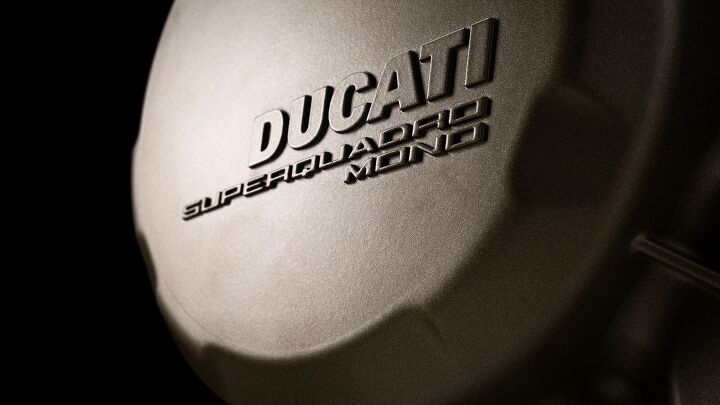The image features a textured, gray plastic cap with evenly spaced indentations and rays around its circumference designed for grip, which facilitates screwing or unscrewing. Prominently displayed on the cap are the words "Ducati" in bold, all-capital letters, with "Superquadro Mono" written beneath it in smaller uppercase font. The background of the photo is predominantly black, with a subtle object resembling a pipe or line visible on the right side of the frame. The lighting highlights the surface of the cap, enhancing its details against the dark backdrop.